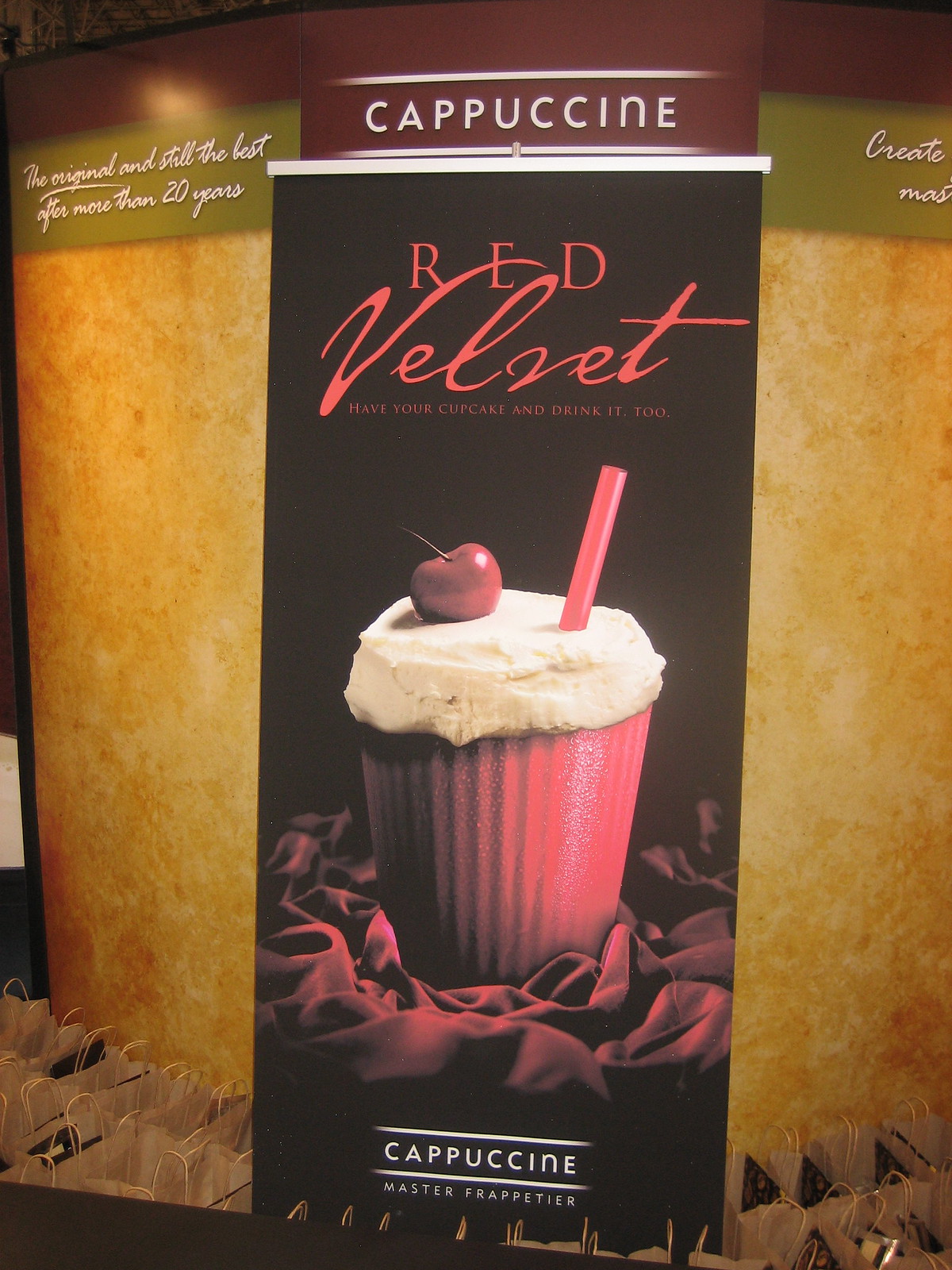The image is a vibrant and colorful advertisement for Capucine, designed to look like a vertical billboard or standing sign, placed in what appears to be an indoor setting against a corner wall. The top of the sign features a maroon background with bold white text spelling "Capucine." Just below this, on a darker brown section with red highlights, the words "Red Velvet" are prominently displayed. Beneath this, in smaller print, the tagline reads, "Have your cupcake and drink it too." 

Central to the advertisement is the image of a drink that closely resembles a cupcake. The drink, likely a frappe, features a red cake-like base topped with whipped cream, a cherry, and a red straw. This cupcake-inspired beverage sits on a slightly crumpled red sheet, enhancing its presentation.

At the bottom of the sign, the phrase "Capucine Master Frappetier" is displayed, tying the theme of the advertisement together. The overall background of the sign is black, and the image is well-illuminated, hinting at a well-lit interior environment. Surrounding the sign are small paper bags, adding to the commercial atmosphere. 

The advertisement hints at a slogan on the top left corner stating, "The original and still the best after more than 20 years," while the top right corner partially displays the word "create." The entire image is lively, well-lit, and clearly designed to draw attention to the innovative red velvet frappe being promoted.